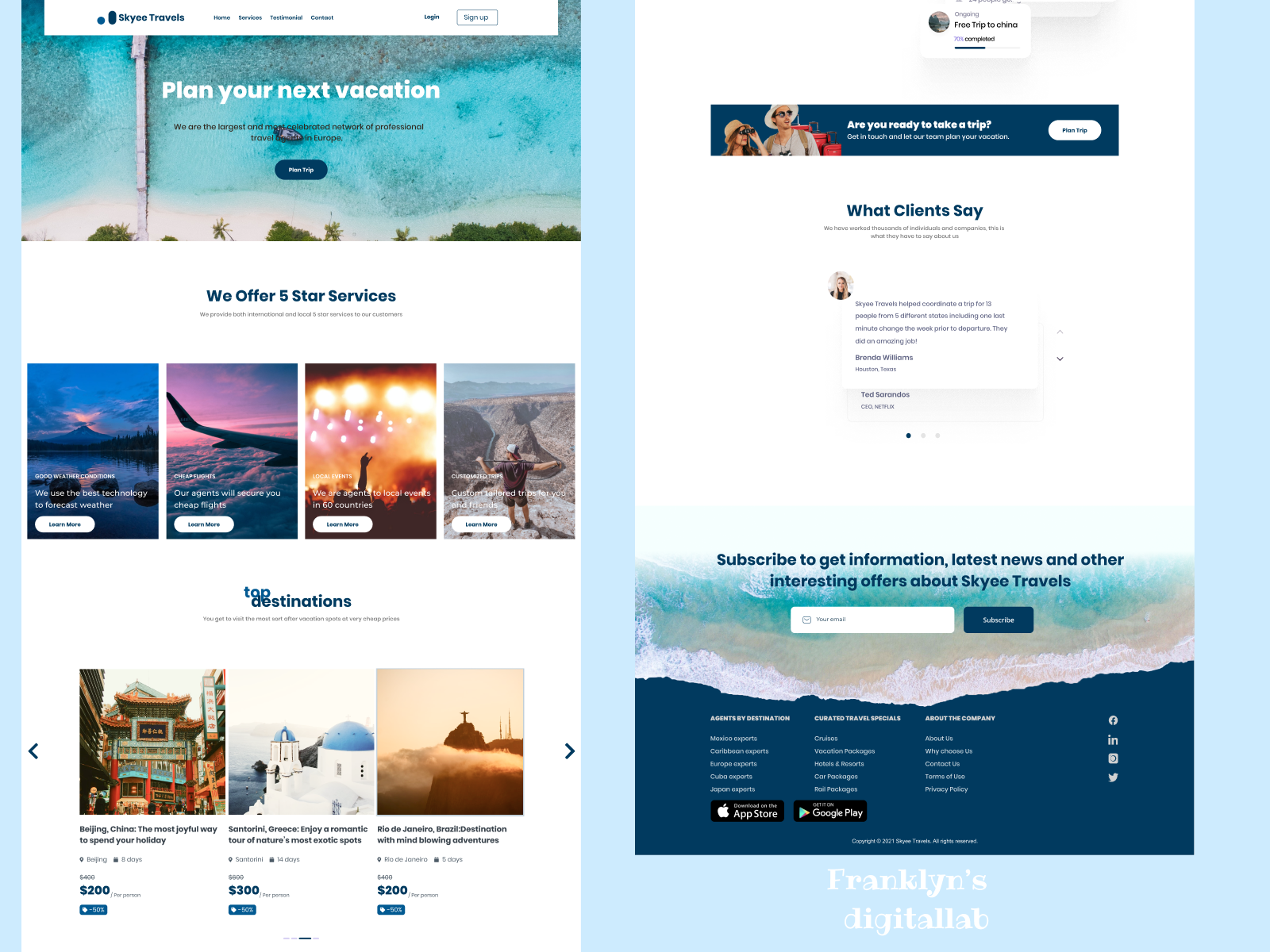An aerial photograph showcases a pristine blue ocean meeting a sandy beach, adorned with the lush green tops of palm trees. At the center of this image, bold white text reads "Plan Your Next Vacation," followed by two rows of smaller black text and a blue bar filled with white text.

Below this image, a white box contains blue text stating, "We offer five-star services," with another indecipherable row of black text underneath. Adjacent to this are four aligned images:

1. A nighttime snapshot of water stretching to the horizon, where a mountain and tree silhouettes stand against a dusky blue sky.
2. A vivid sunset scene captured from the clouds, displaying pink and purple hues with the black silhouette of an airplane wing entering from the right.
3. A concert photograph featuring bright, blurred lights above, and the silhouetted hand of an audience member flashing the rock-and-roll gesture, surrounded by other silhouettes.
4. A man standing on the edge of a dusty canyon, gazing into the distance, wearing a blue handkerchief, a t-shirt, and shorts.

Below these images is a title, "Destinations," with the initial "D" artistically designed as a blue butterfly wing. Following are three more pictures:
1. An Asian-style awning with red posts.
2. A white Grecian building featuring blue domed roofs.
3. A foggy or cloud-covered scene around a mountain topped with a cross or possibly the Brazilian Christ the Redeemer statue.

Further down is a white box with the heading "What Clients Say" in blue text. Above it, a photo of a woman with shoulder-length brown hair in a hat, holding binoculars, stands beside a man wearing circular sunglasses, a white cap, and a backpack. To the right, white text declares, "Are you ready to take a trip," followed by more unreadable white text and a white bar with blue writing.

Underneath, another blue "What Clients Say" heading precedes two rows of black text. To the left is a circle featuring a blonde woman’s picture, followed by eight rows of black text, a blue circle, two gray circles, and finally, a blue section urging, "Subscribe to get information, latest news, and other interesting offers about Skye Travels." The subscription area includes a white search bar and a blue button with white text.

At the bottom, "Franklin's Digital Lab" appears prominently in white text.